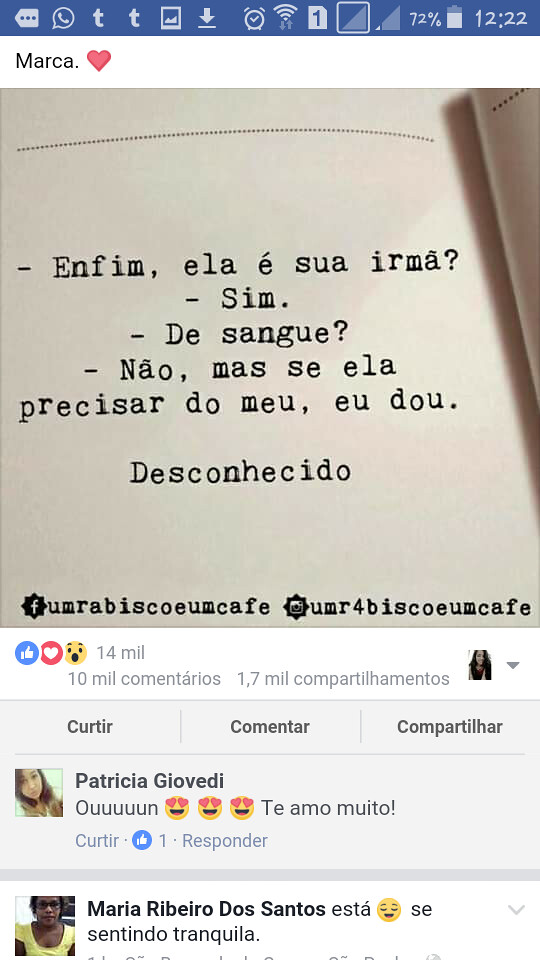This vertically oriented screenshot, taken from a cell phone, showcases a social media post on what appears to be a Spanish version of Facebook. At the top of the image is a blue bar containing several gray icons: three dots on the far left, followed by a phone icon, the Twitter logo, a download button, an alarm clock, a Wi-Fi signal indicator, a "1" in a square, the battery status at 72%, and the time displayed as 12:22. Below the blue bar, there's a white interface with "Marka" accompanied by a red heart icon. 

The main content features an image of a white piece of paper with black text written in a foreign language. Below the post, there's engagement data showing "14 mil" (14 million) alongside icons for thumbs up, a heart, and a surprised emoji. The comments section includes multiple user interactions: one comment from Patricia Giovetti with a heart-eyed emoji stating "te amo mucho," and another from Maria Ribeiro dos Santos expressing that she is "se sentindo tranquila," each accompanied by their respective profile photos.